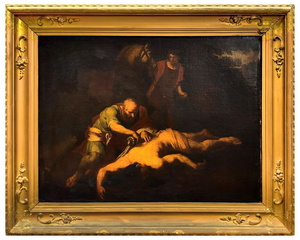This is an image of an antique, Renaissance-style oil painting with a lavishly ornate, gold frame. The frame is thick and intricate, featuring raised decorative elements that enhance its opulence. The painting, though dark and somewhat ambiguous, depicts three individuals. In the foreground, a half-naked figure lies on the ground, potentially unconscious or deceased, their face down on the floor. A second person, dressed in a greenish shirt or robe, leans over the prone figure, seemingly attending to them with a hand placed on their back. In the background stands a third individual, clad in black with a red jacket, holding an object that could be a torch or weapon, their pose and intention remaining unclear. Both standing figures direct their attention towards the person on the ground, adding to the painting's enigmatic narrative. The entire scene is hard to decipher due to the painting's dark tones and lack of explanatory text. The photograph of this painting appears to capture it hanging on a wall with a plain white background.